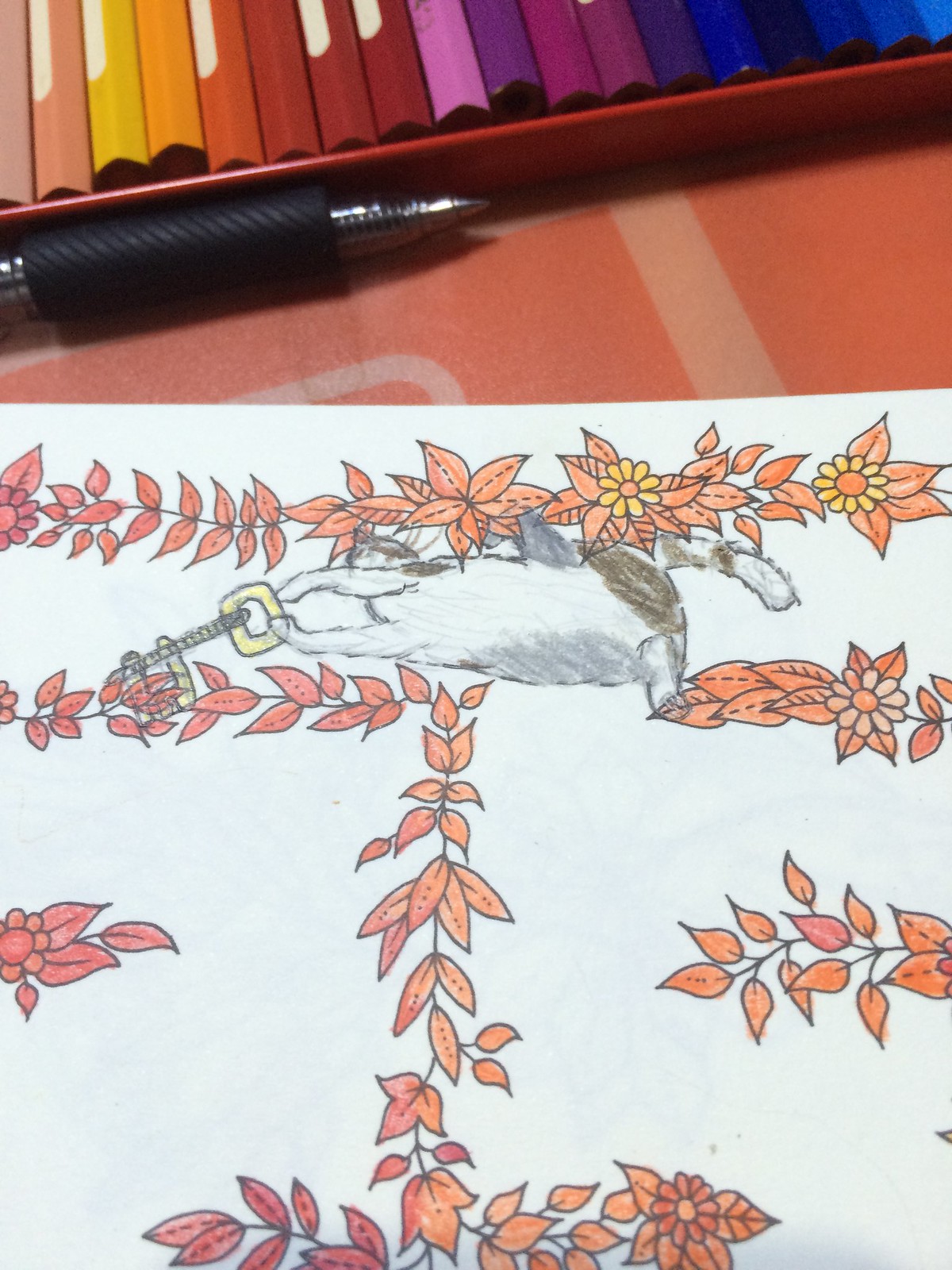A detailed and descriptive caption for the photograph could be:

"An intricately hand-drawn image rendered in various shades of colored pencil. The top portion of the artwork is adorned with a vibrant border of orange, red, and yellow flowers. Below this floral border, a charming cat, illustrated in brown, white, and gray hues, is depicted holding a handsaw with a distinctive yellow handle and a silver blade. The cat appears engaged in the whimsical task of sawing through another layer of the same vibrant orange, red, and yellow flowers, with a flurry of severed flowers gracefully falling below the level. The detailed drawing is set against a stark white background. Above the main illustration, a mechanical pencil rests on an orange surface, hinting at the tools used in the creation process. Additionally, a container brimming with an array of colored pencils can be seen at the top of the image, showcasing the artist’s palette of vibrant colors."